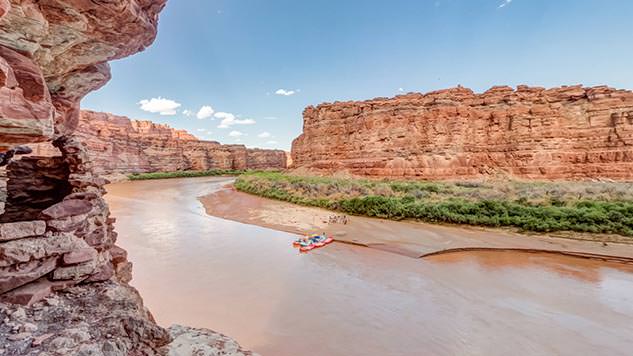This photograph captures a breathtaking landscape that resembles the scenery of Colorado or Arizona, potentially even the Grand Canyon. Dominating the left quarter of the image is a towering rock formation, through which viewers get a peek of the expansive scene beyond. The landscape features a brownish, muddy river that begins at the right side of the photograph, meandering gracefully towards the left edge before curving back to the right. The river is nestled between massive rock cliffs that frame both sides of the image, creating a canyon-like atmosphere.

In the middle ground of the photo, close to the opposite shore, there are small boats—one red and one blue—with faint figures of people nearby. These adventurers appear to have paused their journey on a sandy, rock-strewn beach, surrounded by a lush band of green foliage. The clarity of the bright, blue sky, scattered with a few white clouds, adds to the overall sense of openness and the stark contrast against the rugged, earthy tones of the cliffs and murky river water. The entire scene combines elements of nature's grandeur, serenity, and the human quest for exploration.